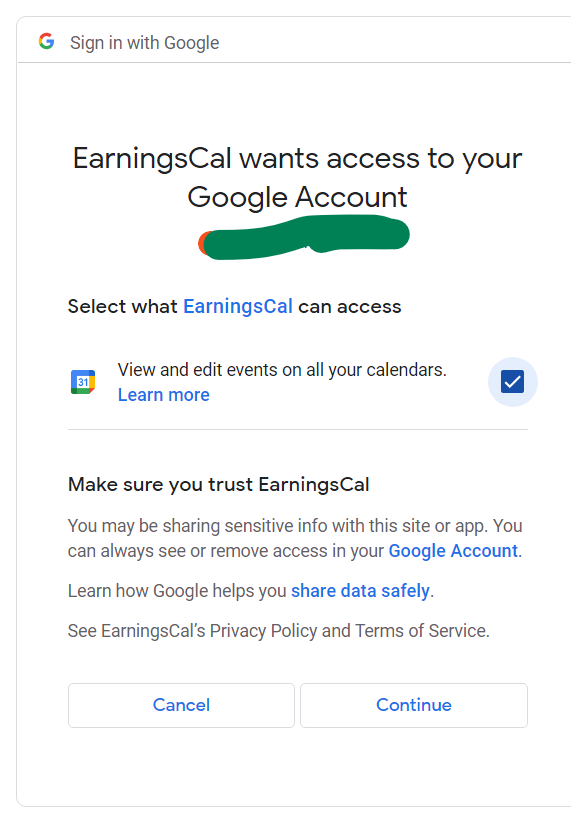The webpage features the Google logo at the top, displaying the iconic "G" in the signature Google colors of red, yellow, green, and blue. Below the logo is the text "Sign in with Google." Centrally positioned on the page, there is a prompt stating, "Earnings Cal wants access to your Google account." The text below this section has been obscured with green marker. 

Further down, it reads, "Select what Earnings Cal can access," where "Earnings Cal" appears in blue text, in contrast to the rest of the sentence which is in black. Accompanying this is a Google Calendar icon featuring the number 31 in the center. This is followed by the statement, "View and edit events on all your calendars," and a link, "Learn more," in blue text. Adjacent to it is a small blue circle containing a checkmark.

The next section advises, "Make sure you trust Earnings Cal," followed by a caution in gray text stating, "You may be sharing sensitive info with this site or app. You can always see or remove access in your Google Account," with "Google Account" in blue text. Additionally, it mentions, "Learn how Google helps you share data safely," with "share data safely" also in blue. Following this, there is a link to "See Earnings Cal's privacy policy and terms of service."

Two buttons are located at the bottom of the page, outlined in gray. The first button, labeled "Cancel," and the second, labeled "Continue," both feature blue text.